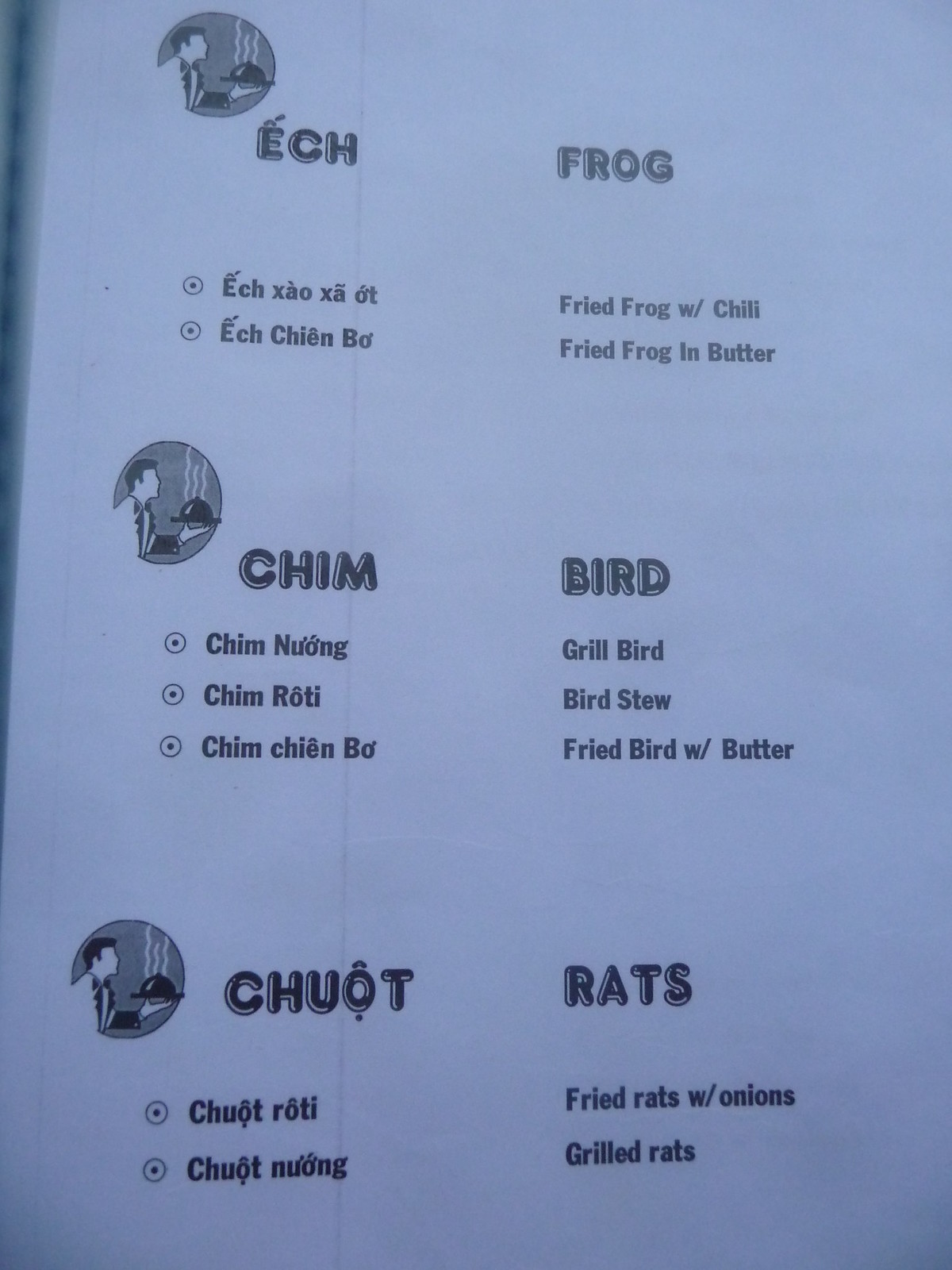This photograph appears to be a snapshot of a menu, specifically the back page which features a light grayish-white background. At the top, there is a small cartoon image of a man serving a tray, which is repeated at various sections throughout the page. On the left side of the menu, there are entries in a different language, possibly Vietnamese, and their corresponding English translations are listed on the right.

At the top left corner, the menu lists "ECH" with "frog" written beside it in English. The translated items include:
- "ECHXAOXAOT," which is described in English as "fried egg with chili."
- "Fried frog in butter."

Further down the menu, the next section starts with the cartoon picture and the word "CHIM," which is translated as "bird" in English. The items under this section are:
- "CHIM NUNG," which is translated to "grilled bird."
- "Bird stew."
- "Fried bird with butter."

The final section also features the man serving a tray and the word "CHUOT" which is translated as "rats" in English. The items listed here include:
- "Fried rats with onions."
- "Grilled rats."

This menu provides a glimpse into a unique culinary experience, showcasing a variety of exotic dishes alongside whimsical cartoon imagery.